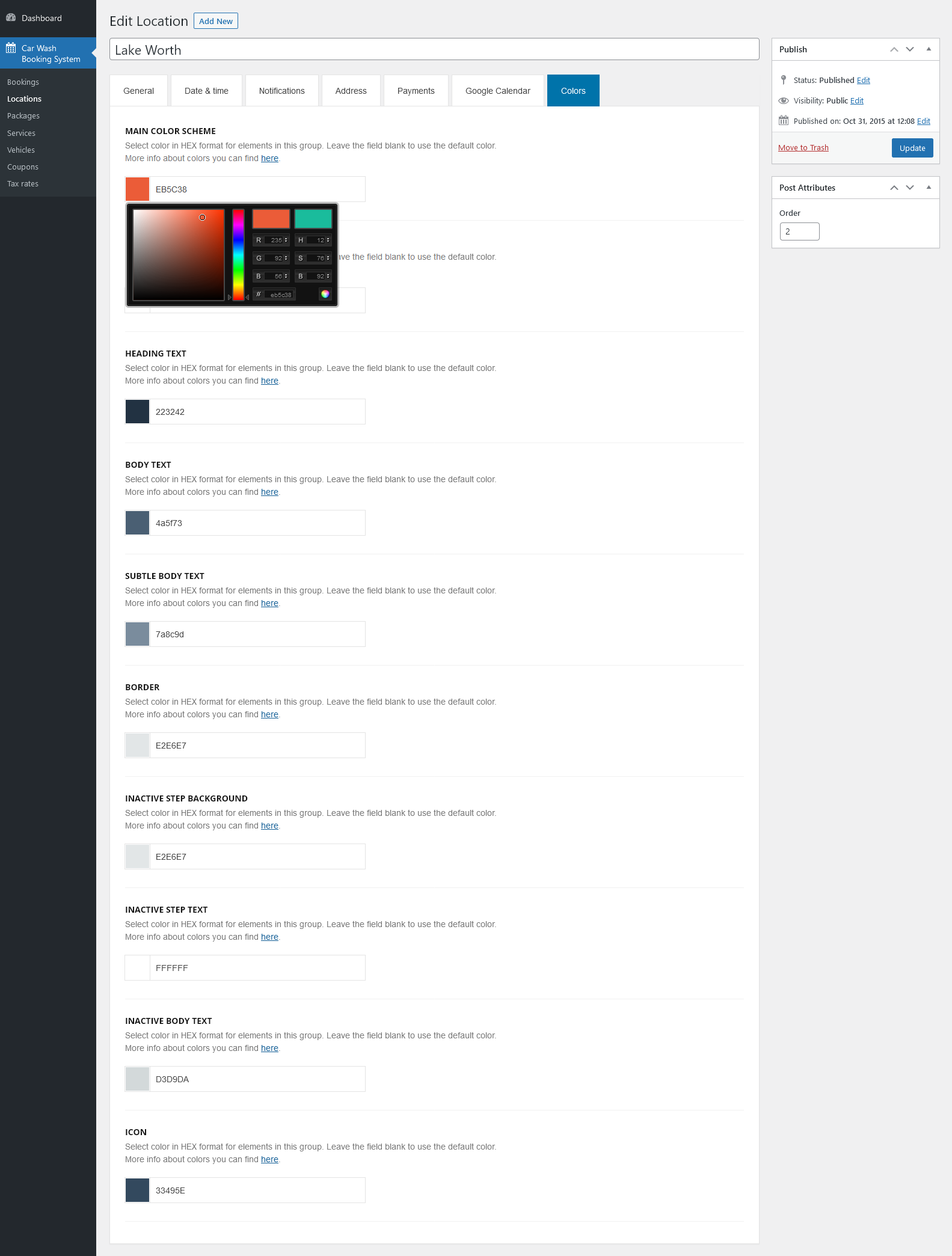**Detailed Caption:**

This image showcases the settings tab of a website. On the left side, there is a vertically arranged navigation dashboard with various options. The dark gray color of the navigation bar contrasts with the lighter gray of the main content area, where the text appears quite small. 

To the right, a light gray box features prominently at the top, with headings such as "Edit Location" and "Add New." Below these headings, the location "Lake Worth" is displayed. Several tabs are also visible here, labeled "General," "Date and Time," "Notifications," "Address," "Payments," "Google Calendar," and "Colors," with the "Colors" tab highlighted in blue, indicating it is currently selected.

The section under the "Colors" tab includes options to customize the main color scheme of the site using a color grid and sliders. Specific settings for various text and design elements are listed, such as "Heading Text," "Body Text," "Subtle Body Text," "Border," "Inactive Step Background," "Inactive Step Text," and "Inactive Body Text Icon."

On the right side of the page, there is a lighter green section containing publishing options. It includes buttons and fields for "Publish," "Publish Status," "Publish Edit," "Visibility," and the publishing date, marked as "October 21st, 2015." Additional options like "Move to Trash" and an "Update" button are also present. Below these, attributes such as "Post Attributes" and "Order" are displayed within this green-colored section. The entire interface maintains a clean, organized layout with a white background for the color selection box.